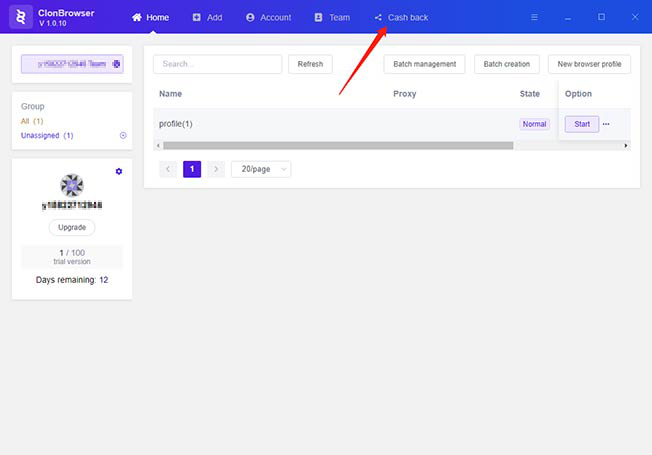The image displays a software application interface, likely running on either a tablet or a desktop PC, suggested by its aspect ratio. The application is named "Clone Browser," as indicated by a blue banner at the top, and is identified as version 1.0.10 on the left side of the banner. The interface's Home panel is currently selected and displayed as slightly grayed out. Adjacent to the Home panel, there are navigation tabs labeled Add, Account, Team, and Cashback. Additionally, typical window control icons—Minimize, Maximize, and Close (X)—are located in the top-right corner.

Beneath the top banner, there are several interface sections. On the far left, three small vertical panels are displayed. The topmost panel features a blue button with fuzzed-out text, suggesting obscured or redacted identifying information. Below this button, the panel lists options labeled Group, All, and Unassigned, with "All" marked in red and "Unassigned" in blue. Further down, more grayed-out text is visible, indicating more redacted content, along with an "Upgrade" button. This section also mentions that the user is on a trial version of the application, with "Trial Version 1 out of 100, Days Remaining 12" displayed, implying a shareware model.

To the right of these small panels, the main section of the interface features a large, predominantly white panel. At the top, there is a search bar followed by a refresh button and three additional buttons labeled Batch Management, Batch Creation, and New Browser Profile. Below these buttons, "Profile 1" is shown in parentheses as the name of the profile, accompanied by an Options button and a blue Start button. Despite the interface having the capacity to display up to 20 pages of profiles, currently, only one profile is listed, indicating a single page in view.